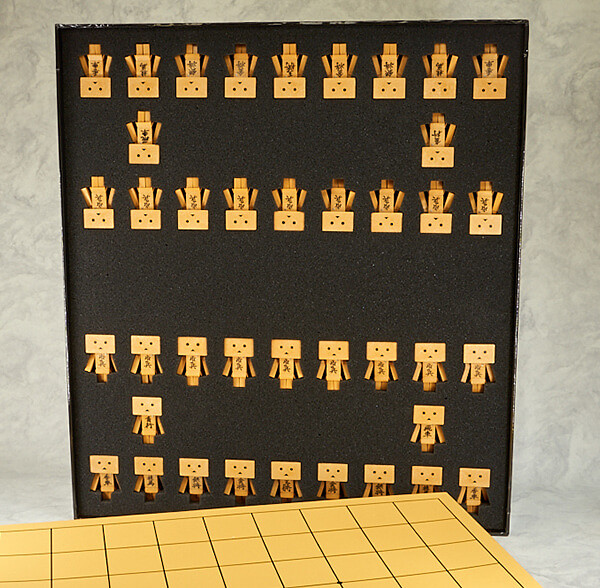The image shows a black board adorned with square-shaped characters resembling figures from a video game like Minecraft. These figures have square heads with dots for eyes and open mouths that form a somewhat sad expression. They also have rectangular bodies and limbs. The characters are uniform in their beige to yellow-orange color and each has what appears to be Japanese kanji on their chests. Arranged in several rows, the top rows of characters are upside down while the bottom rows are right side up. The board itself has a texture or pattern that includes foam to situate the figures snugly. The background appears to be a white marble-like wall, giving an elegant contrast to the playful and structured arrangement of the square figures.